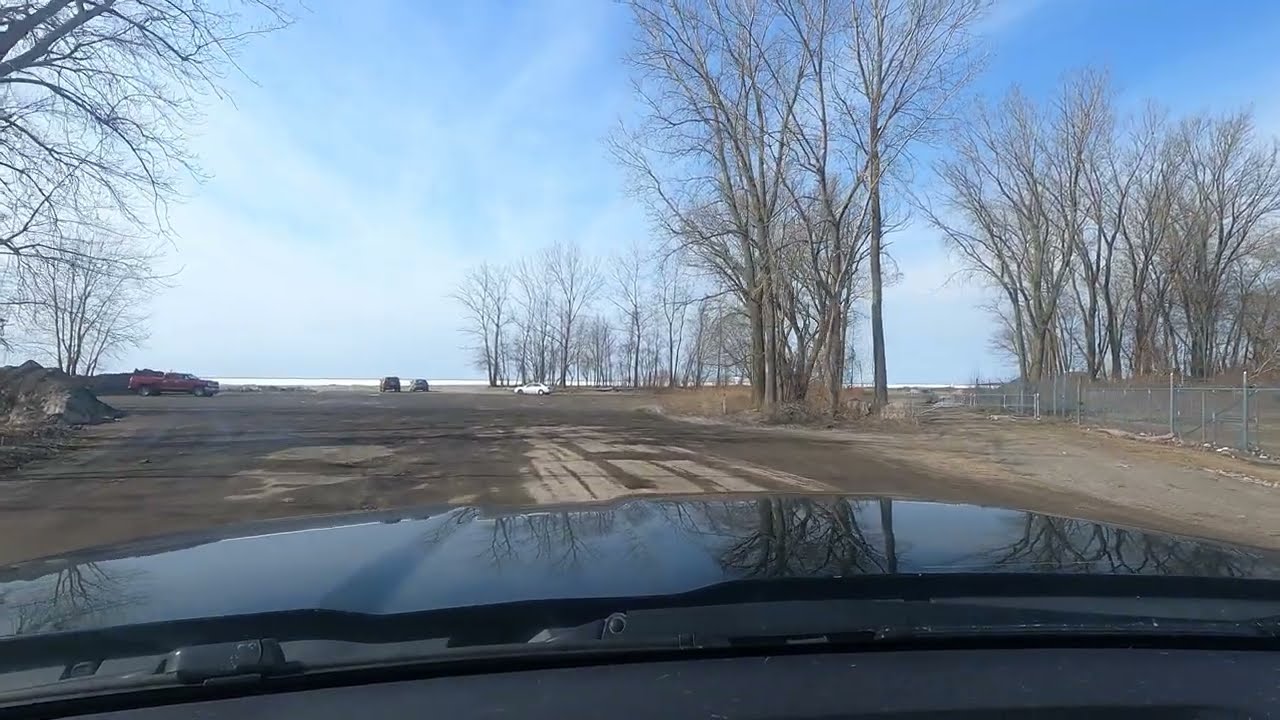The image is a color photograph in landscape orientation, viewed through the windshield of a car. The foreshortened black hood and windshield wipers dominate the bottom half of the frame. Through the windshield, a vast, bare dirt parking lot stretches out, looking muddy in places with varying shades of brown, possibly indicating wet and dry patches. The lot is empty except for the car from which the image is taken. On either side of the lot and bordering the scene are leafless, presumably dead trees, creating a stark, wintry atmosphere. To the right side, a chain-link fence is visible, adding to the barren look of the surroundings. In the far distance, near the horizon, several vehicles are parked amidst a line of trees. The sky above is mostly blue with streaky white clouds, darker in some areas, providing a serene yet somewhat desolate backdrop to the scene.